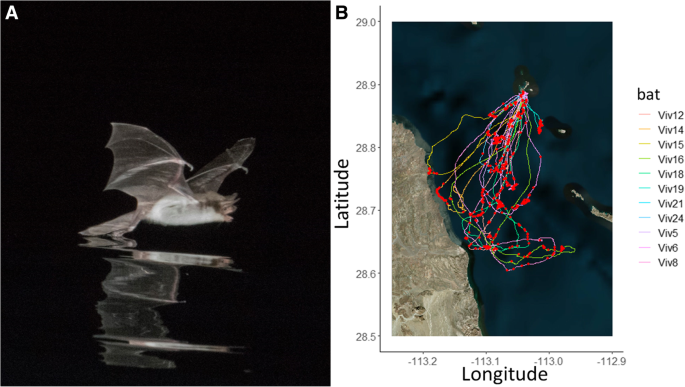This detailed infographic illustrates the flight patterns and migration data of bats. The left side features a striking photo of a bat in flight over a body of water, its reflection visible against a dark black background. The bat is primarily brown with a lighter, white belly. 

On the right, an aerial map is overlaid with a detailed XY graph, where the y-axis ranges from 28.5 to 29 in latitude and the x-axis from -113.2 to -112.9 in longitude. This map highlights a grayish-brown landmass in the lower left corner and surrounding ocean with smaller islands of similar appearance. Multiple colored pathways in purple, green, yellow, and blue indicate different flight paths, dotted with red points marking specific locations.

The flight paths, resembling a large teardrop shape, suggest migratory routes of bats tagged with GPS locators. Labels such as VIV12 to VIV24 enumerate eleven distinct flight paths on the right side of the map, showcasing the extensive tracked movement of these bats.